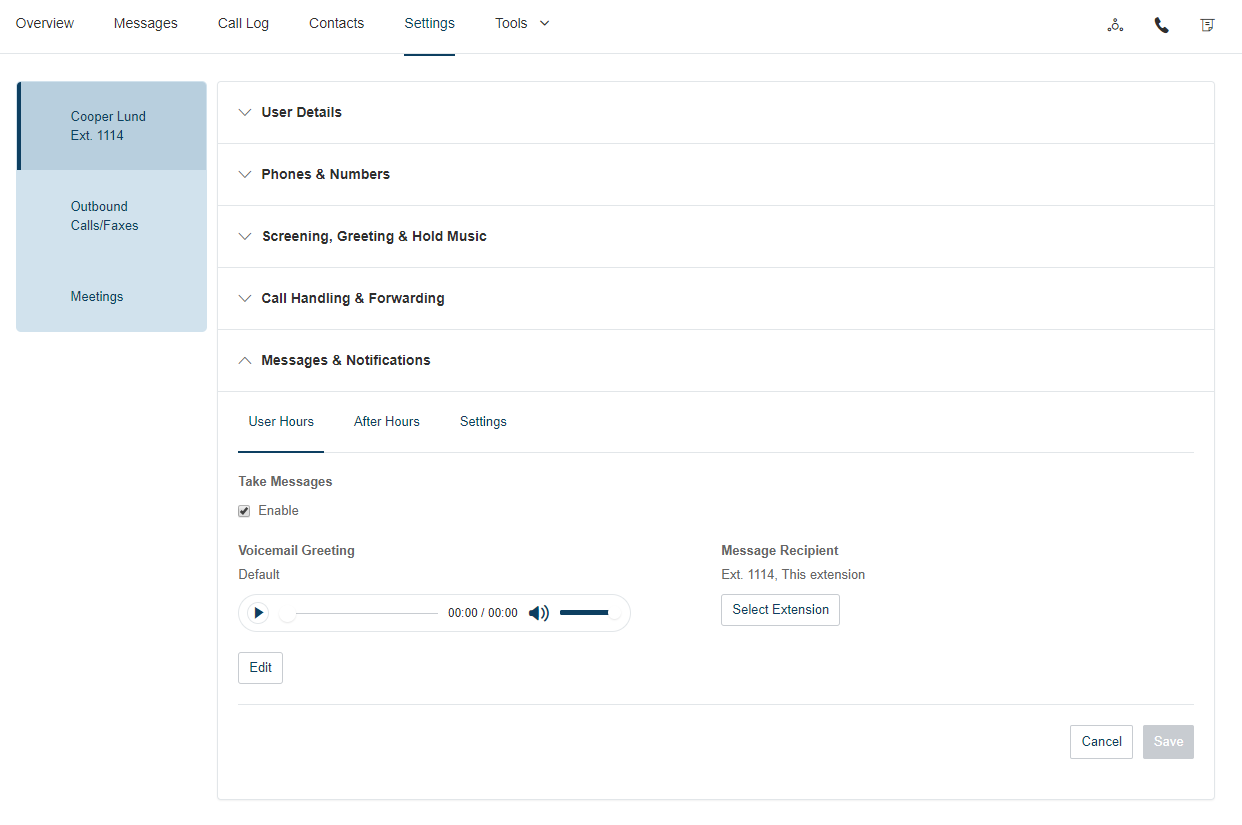The image displays a detailed interface of a communication or call management application. At the top, there's a light blue header labeled "Cooper Line, ext 1114," indicating an outbound call. The interface includes several sections such as:

- **Overview, Messages, Call Log, Contact Settings, and Tools:** These sections likely provide different functionalities for managing calls and messages.
- **Navigation Icons:** A circular icon with three smaller circles around it, a phone icon, and an icon resembling a receipt.
- **Settings Menu:** The "Settings" option is underlined, indicating the current selection.
- **Left Sidebar:** Features options like "Call/Boxes," "Meetings," and "User Details," each accompanied by drop-down menus for expanded choices.
- **Options within Settings:** The settings menu includes:

  - **Phones and Numbers**
  - **Screening, Greeting, and Hold Music**
  - **Call Handling and Forwarding**
  - **Messages and Notifications**
  - **User Hours (currently underlined)**
  - **After Hours Settings**

- **Take Messages Section:** This section seems to allow enabling voice mode:

  - **Enable Voice Mode:** An option with a check mark indicating it's activated.
  - **Default Greeting:** A setting that can be toggled with options for playback labeled "0000" for full speaker message.
  - **Recipient Info:** Shows details for recipient "ext 1114" tied to the specific extension.
  
- **Action Buttons:** 

  - **Select Extension:** A rectangular button.
  - **Edit:** A centrally placed square button.
  - **Dotted Line Separation:**
  - **Cancel:** A square button.
  - **Save:** A gray square button.

The background of the entire interface is white, giving it a clean and clear display for various settings and options.